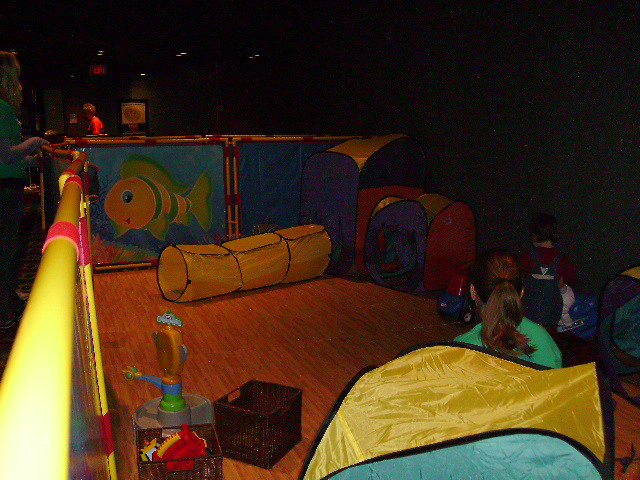This photograph, though dimly lit, vividly captures a children's play area within a large, somewhat darkened room. Central to the scene is a rectangular play zone, approximately 15 feet by 10 feet, enclosed by a child-friendly barrier made of colorful plastic tubes—red, yellow, and purple. The barrier features cheerful, child-themed decorations, including a prominent yellow and green striped cartoon fish with a solid yellow face and green fins. Within this fenced area, the orange floor is scattered with various toys, suggesting a space bustling with play.

A toddler, donned in blue overalls and a long-sleeve red shirt, stands with their back to the camera, positioned towards the right side of the frame. Nearby, a woman with a brown ponytail, clad in a green shirt, appears to be tending to the child. The backdrop includes a wall adorned with the cartoon fish and possibly other whimsical designs. Additionally, a yellow, flimsy tunnel, likely a play contraption, stands out as a feature meant for children to crawl through.

In the foreground, to the left, there's a brown basket, seemingly empty, next to which lies a small plastic figure with a blue shirt and green ear. This basket likely serves as storage for the scattered toys. The overall scene is one of playful vibrancy amid darker surroundings, capturing the essence of a lively play space designed for young children.